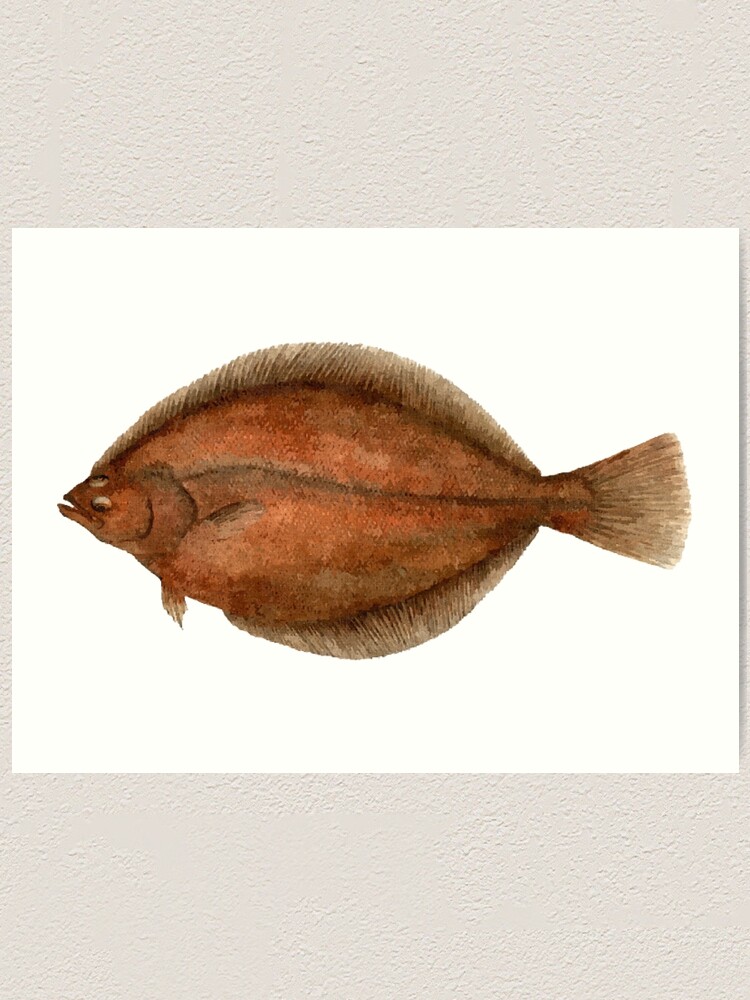The image is of a photograph or drawing depicting an ancient-looking fish, set against a textured white background, reminiscent of stucco. The fish is positioned on a rectangular white piece of paper. Its body is short and very rounded, featuring a mix of orange, amber, and brown hues, with a distinctive brown line running down the center towards its tail. The fish has long fins extending the entire length of its body both top and bottom; the upper fin stretches from its nose to the tail, while the lower fin starts midsection and extends to the tail. The fish has a very tiny face and snout, with two visible eyes – one on top of its head looking upward and another below it, looking downward. This side-profile depiction of the fish appears flattened, adding to its unique appearance.